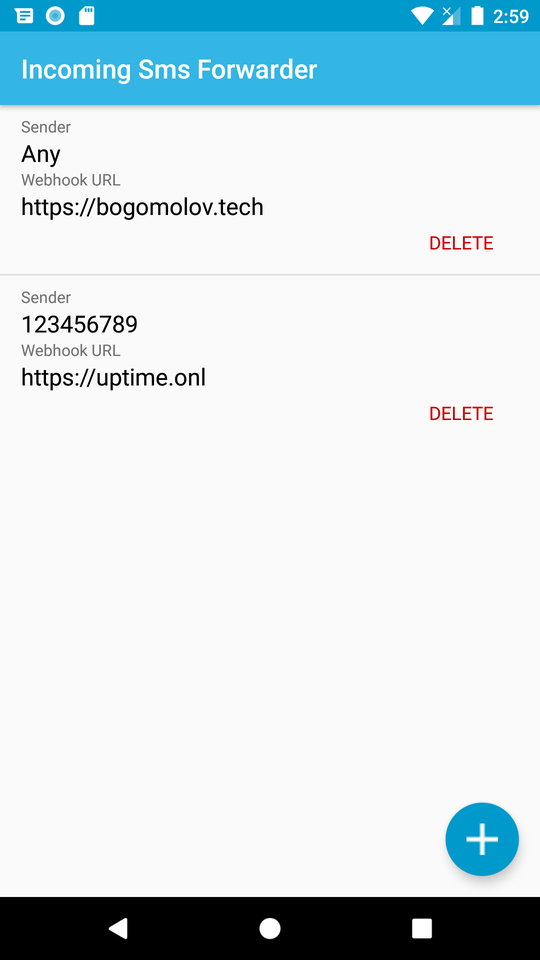This is a detailed screenshot from a mobile phone. At the top, there is a medium blue status bar displaying various information. Starting from the right, the time is shown as 2:59. Next to the time, there is a fully white battery icon, indicating full charge. Following the battery icon, there is a mobile signal icon that is half filled with a little white 'X' above it, suggesting no active network connection. Next, there is a fully white Wi-Fi icon indicating a strong Wi-Fi connection. After that, there is a white SD card icon, and then a white circle with a blue center. Finally, on this blue bar, there is a small document icon.

Below this status bar is a lighter blue bar with white text that reads "Incoming SMS forwarder." Beneath this, there is a white screen with black text. The first line of text reads: "Sender: any," followed by "Webhook URL: https://bogomolov.tech." In the lower right of this text, there is a "Delete" option in red font. Below this, a black line divides the screen. Following the black line, the text reads: "Sender: 123456789," followed by "Webhook URL: https://uptime.onl."